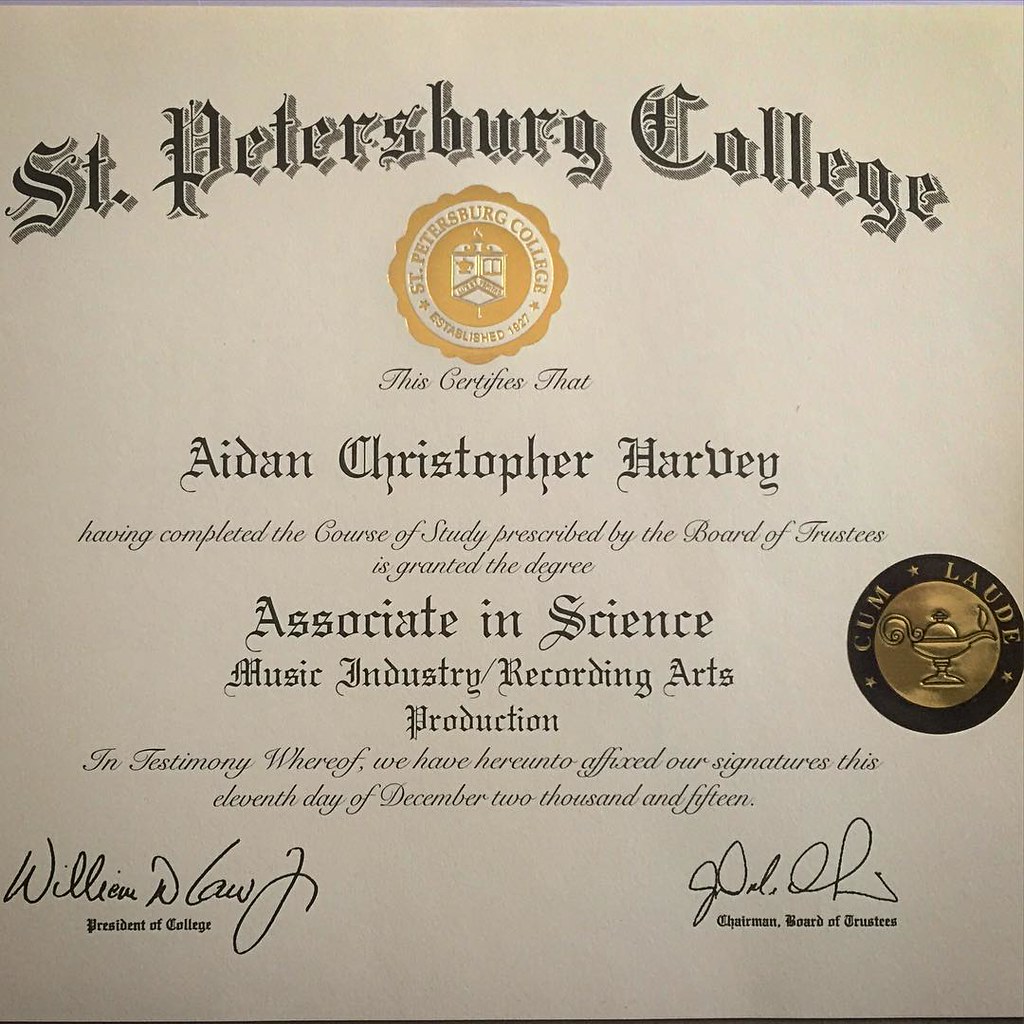The image depicts a detailed and official diploma from St. Petersburg College, awarded to Aidan Christopher Harvey. The diploma certifies that Aidan Christopher Harvey has completed the prescribed course of study and is granted the degree of Associate in Science, specializing in Music Industry Recording Arts Production. The document is dated December 11, 2015, and features two signatures—one from the president and the other from the chairman of the Board of Trustees. Both signatures are affixed at the bottom, although the names are not clearly legible. The diploma includes an official stamp located between "St. Petersburg College" and "this certifies that," with the text "St. Petersburg College, established 1927." Additionally, there is a stamp indicating that Aidan graduated cum laude. The document is visually presented in white, yellow, black, and blue colors.